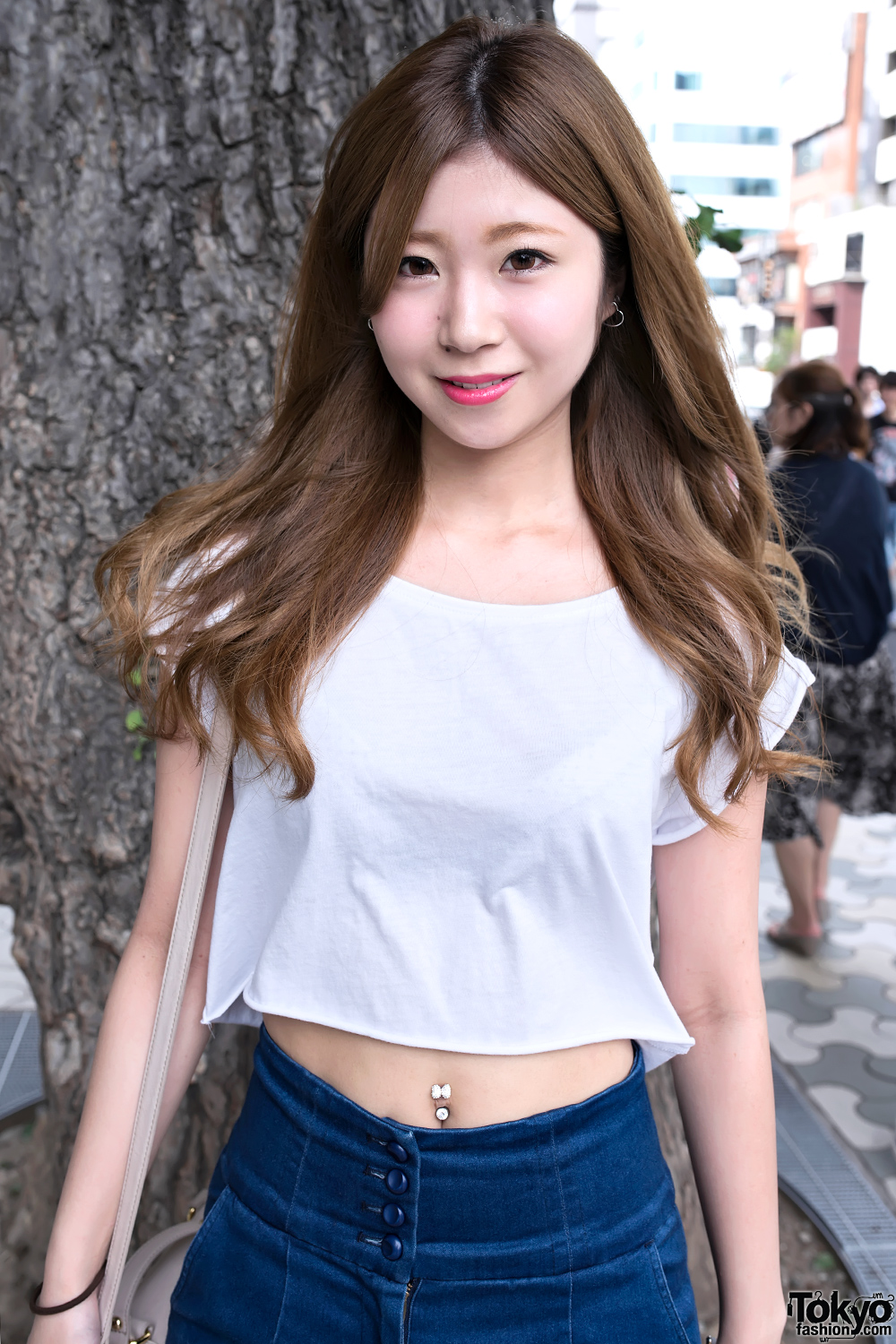This is a close-up shot of a petite Japanese girl standing in an urban setting. She has very long, reddish-brown hair with lighter ends that slightly curl at the tips. Her striking makeup includes hot pink lips and subtle eye makeup. She sports a white short-sleeve crop-top t-shirt that reveals her pierced belly button, adorned with a piece featuring a bow and jewel. She is wearing a tight, high-waisted denim skirt with four buttons in the front. A cream-colored handbag hangs from her left shoulder, while a black hair tie encircles her wrist. Tiny earrings and a leather bracelet on her right wrist accentuate her look. She stands confidently before a large, thick tree, its bark visible behind her. The backdrop reveals a bustling cityscape with people walking on a tiled walkway, large buildings towering above, and additional details like a girl in a black top and skirt in the distance. The bottom right corner of the photograph is marked with “tokyofashion.com," indicating the scene's fashionable urban context.